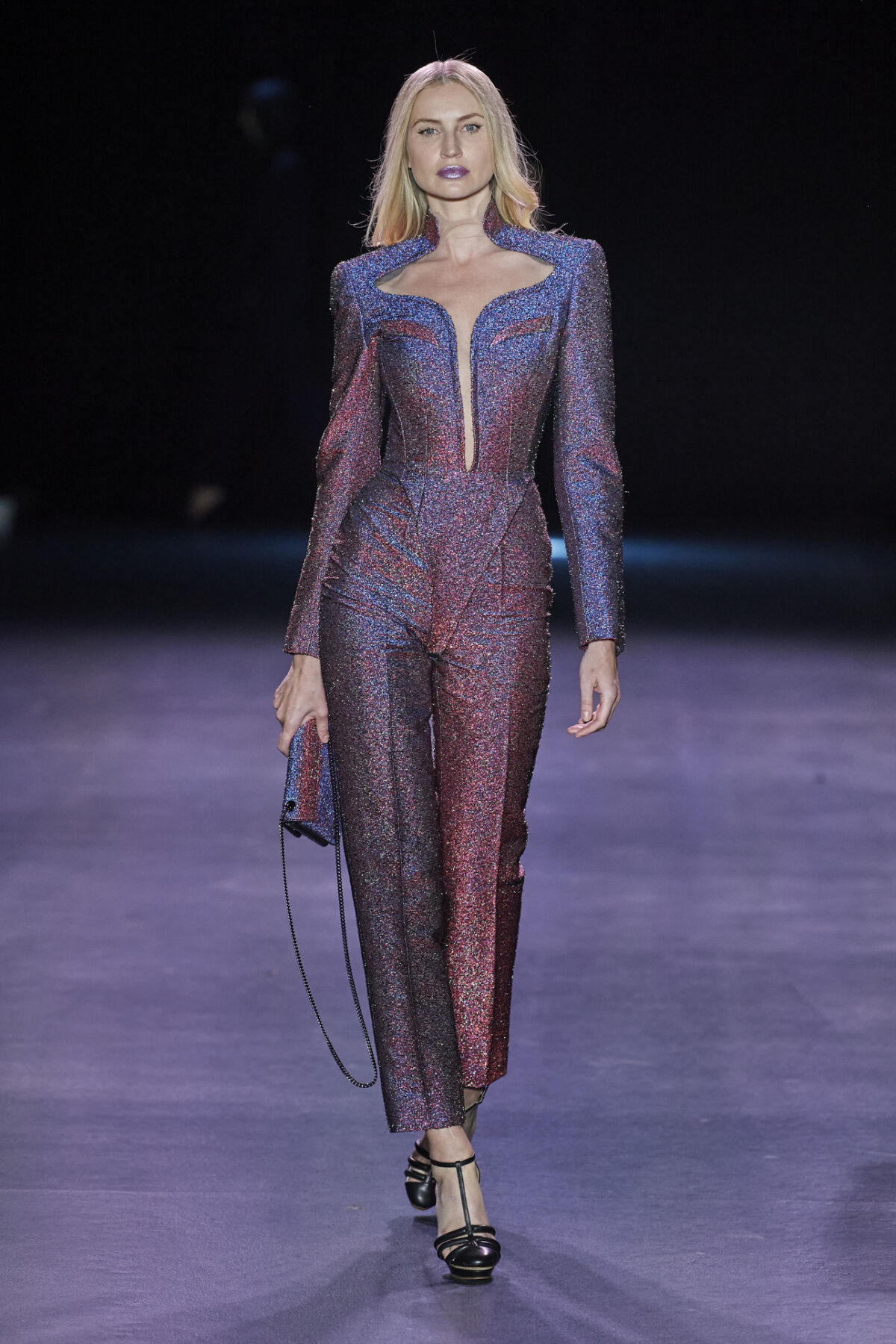In this striking runway scene, a model with long, shoulder-length blonde hair and wearing purple glitter-like lipstick struts confidently under the spotlight. The stage beneath her is a deep purple, contrasting starkly against the completely black backdrop. A barely visible silhouette appears in the background, adding a sense of depth to the composition. 

The model is dressed in a form-fitting, glittery jumpsuit that showcases a mesmerizing gradient from bluish or purplish at the top to reddish at the bottom. The jumpsuit features long sleeves and a dramatic cut-out from the chest down to the belly button, revealing her pale skin in a pronounced V-shape. The design emphasizes her waist with a high-waisted cut, transitioning to looser pant legs. Notably, the right leg of the jumpsuit is a vivid red, while the left leg is a deep blackish-purple.

In her right hand, she holds a coordinating purse that mirrors the glittery color scheme of her outfit, and her ensemble is completed with sleek black heels.